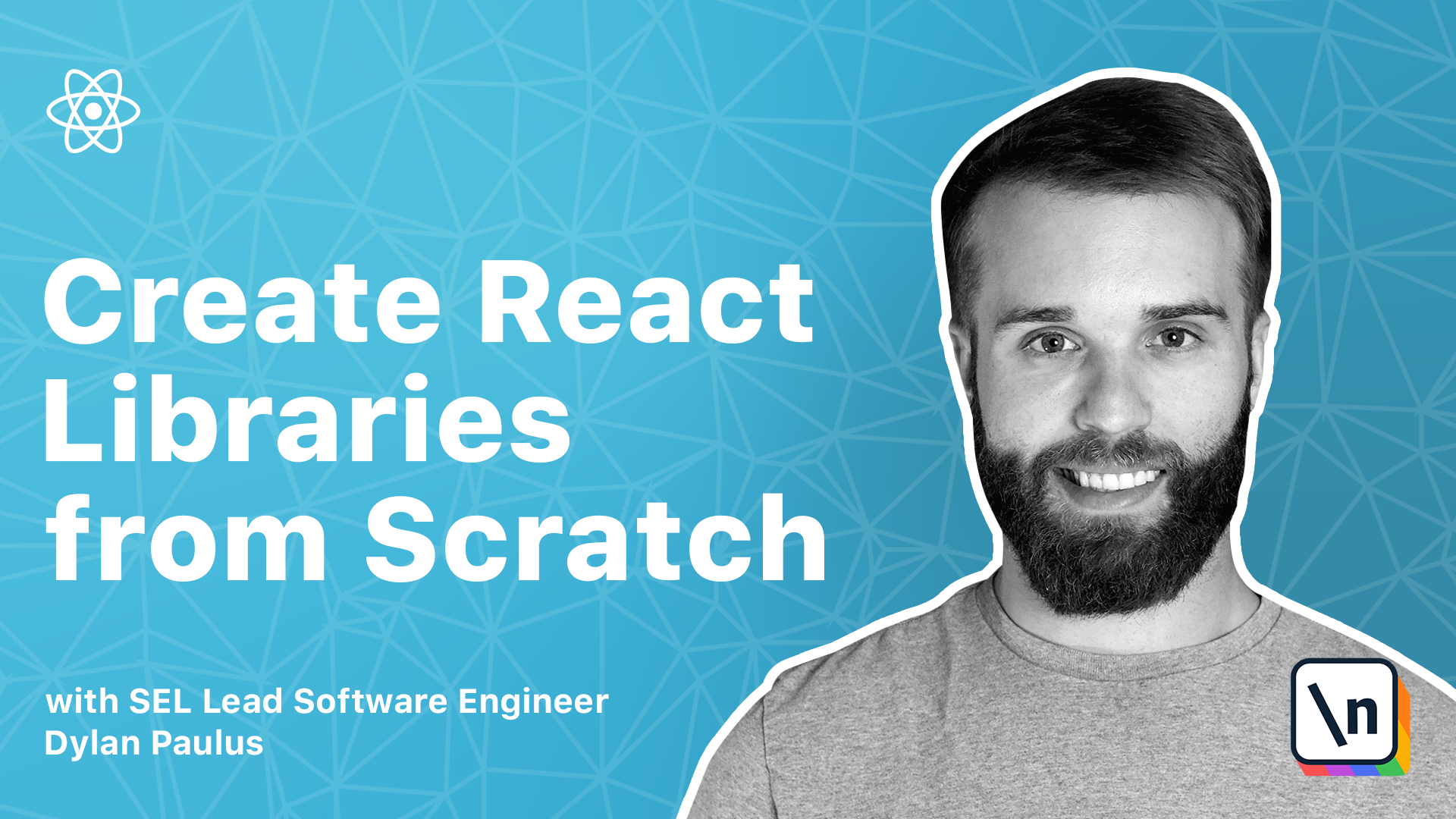The image appears to be an advertisement for a company, prominently displaying a promotional message against a gradient background that transitions from very light blue in the upper left corner to a slightly darker blue towards the right. In the upper left corner, there's a white logo resembling an atom with three electrons encircling it. Just below this logo, a bold, white, almost block-style font reads, "Create React Libraries From Scratch."

Below this main headline, in significantly smaller text, it says, "with SEL Lead Software Engineer Dylan Paulus." To the right of this text, there's a black and white photo of a smiling Dylan Paulus, who has a well-trimmed beard and appears to be wearing a gray t-shirt.

Additionally, there is a symbol present in the image. It is a square with rounded corners, featuring a black trim and a white interior that contains a diagonally positioned black shape and a small "N." Surrounding the square are rainbow colors, adding a distinctive visual element to the ad.